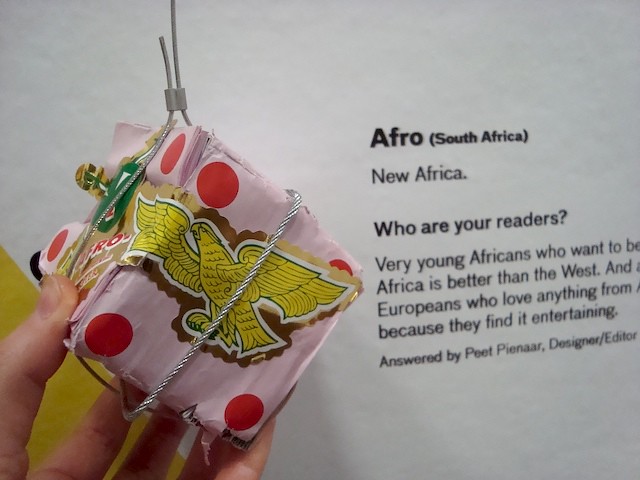The image reveals a small cube adorned in light pink paper with scattered red polka dots, delicately wrapped in silver wire. Atop the cube is a prominent sticker depicting a yellow-golden bird, likely an eagle, set against a gold cutout with a scalloped edge. This ornate box is cradled in a light-skinned individual's hand, their fingertips visible. Positioned to the right of the box, black text on a white background reads: "Afro (South Africa). New Africa. Who are your readers? Very young Africans who want to be. Africa is better than the West, and Europeans who love anything from [cut off] because they find it entertaining." The attribution at the bottom credits Pete Pienaar, designer, and editor.